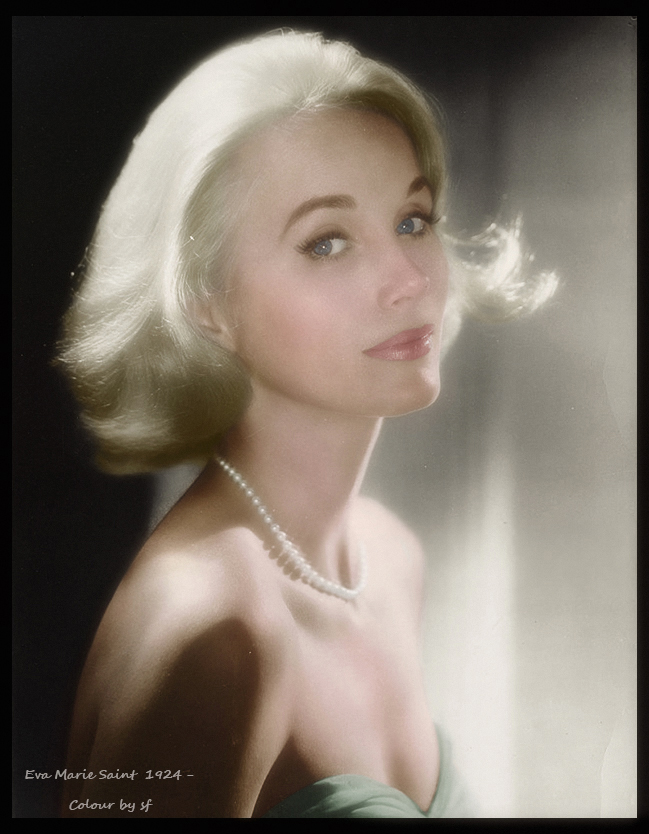This is a beautifully rendered and colored-upgrade image of the famous actress Eva Marie Saint, originally taken in 1924. The photograph, now in color thanks to SF, features a striking white woman with silky, smooth blonde hair just above shoulder length. Her blue eyes and red lips stand out, accompanied by subtle, unobtrusive makeup that enhances her delicate facial features. Eva is adorned with a pearl necklace and is wearing a strapless green dress, which complements her elegant appearance. The background is minimal, with a light source illuminating her from the right, casting the left side in shadow. The clarity of the image suggests it is a high-quality rendering likely found on a modern website. The “colored by SF” note is visible at the bottom left-hand corner of the photo. Despite her serene and somewhat vulnerable expression, Eva Marie Saint exudes a timeless beauty and grace in this photograph.